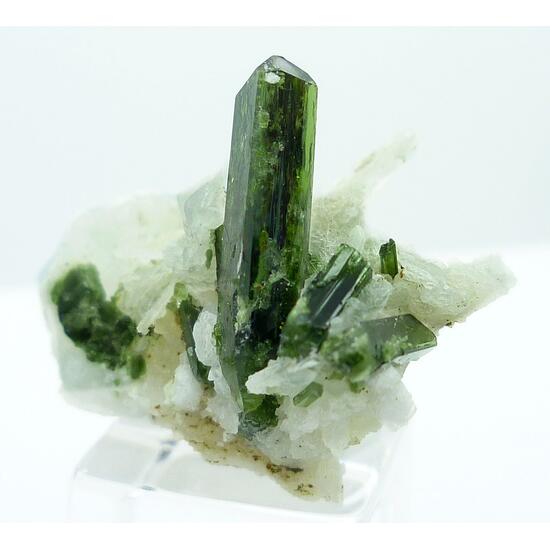The image features a single object, perfectly centered and showcased against a clean, light blue background. This object appears to be a unique rock formation or mineral specimen, characterized by its striking visual details. At its base, there is a rough, white, and somewhat messy structure, interspersed with beige elements. Rising prominently from this base is a smooth, elongated, and slightly pointy cylinder with a translucent, shiny green hue, reminiscent of jade or a green beer bottle. Surrounding this main cylinder, numerous smaller green gem-like formations are embedded within the white crystalline matrix. The lack of text in the image allows the viewer to fully appreciate the intricate and varied shades of green, white, gray, and beige, hinting that this might be a prized find from an archaeological expedition or a rock collector's treasure.